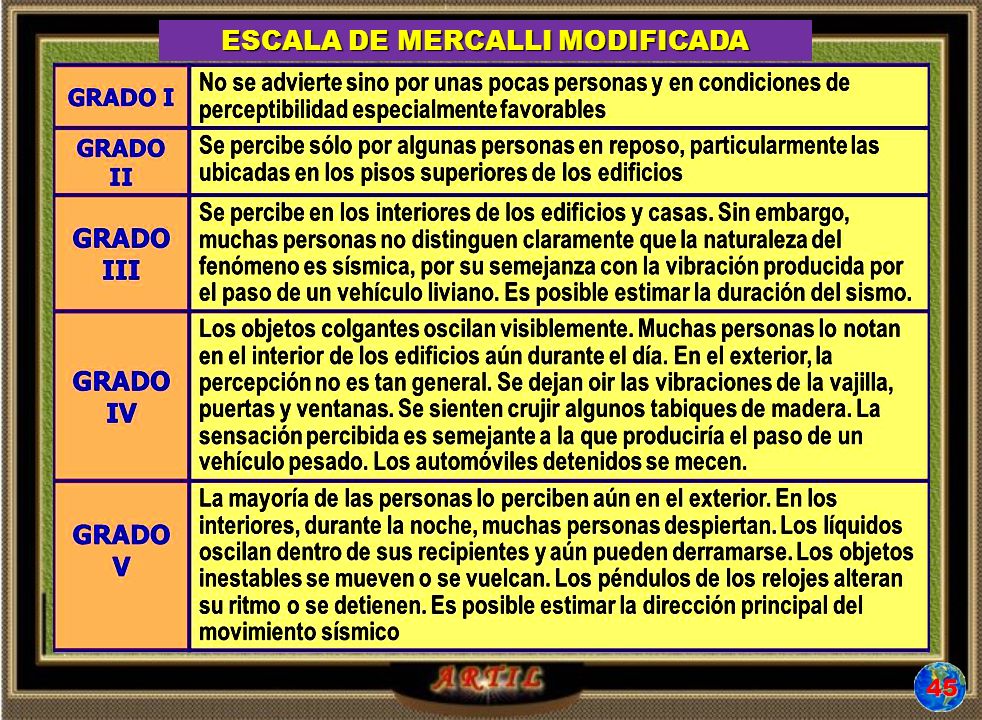The image depicts a detailed table written entirely in Spanish, likely featured as a slide in a PowerPoint presentation. The table is bordered by a green rectangle and has a black border around the outer edge. At the top, the main title reads "Escala de Mercalli Modificada" inside a purple section with yellow lettering. The left column of the table features different grades listed from I to V (Grado 1 through Grado 5) in Roman numerals, each within an orange box with black lettering. Adjacent to each grade is a description written in black lettering on a yellow background, detailing the extent of noticeability and effects of each grade. The image is sectioned into this organized format, and in the bottom right-hand corner, there is a small globe icon with the number "45" inside it in red. The word "artil" is partially visible at the bottom, adding to the distinct elements of this educational slide.